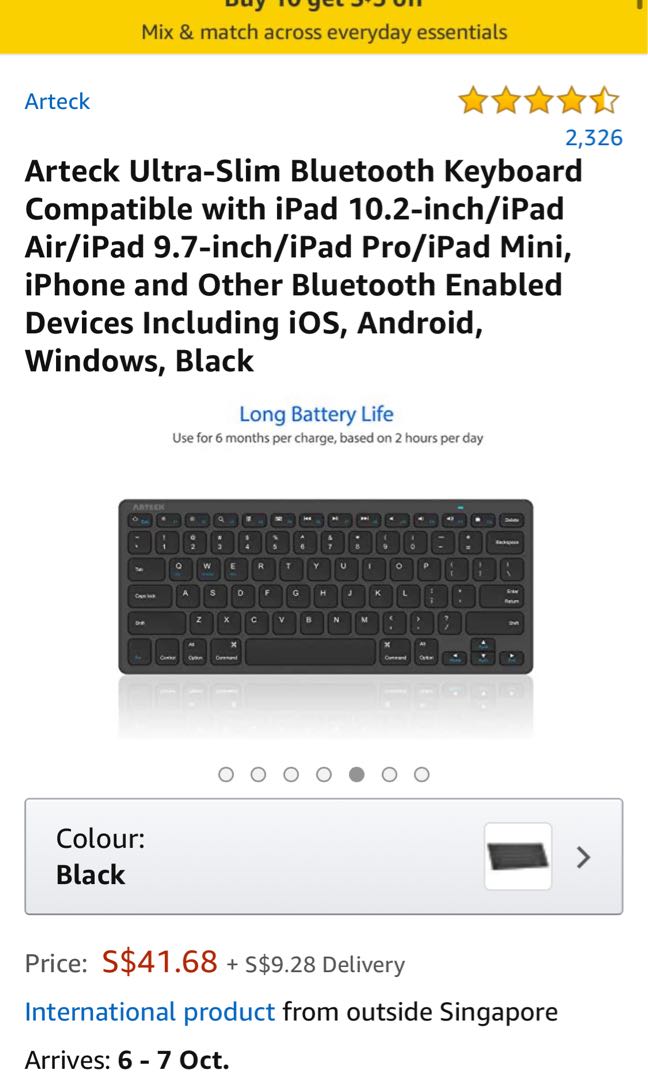The image captures a screenshot from a cell phone, focused on promoting a tech product. At the top of the screen, there's a yellow header with partially cut-off text, but the visible portion reads, "Mix and Match Across Everyday Essentials." Below this, in blue print, the header says "Our Tech" and proudly displays a rating of four and a half stars out of five, visually represented by a row where four and a half stars are colored in yellow. The rating number 2326 is highlighted below in blue.

The featured product is described in black text as the "Our Tech Ultra Slim Bluetooth Keyboard," compatible with a variety of Apple products including iPad 10.2 inch, iPad Air, iPad 2.7 inch, iPad Pro, iPad Mini, iPhone, and other Bluetooth-enabled devices across iOS, Android, and Windows platforms. 

An image of the keyboard follows, showing its sleek, black design. Emphasizing its longevity, blue text states: "Long Battery Life: Use for six months per charge based on two hours per day." The price of the keyboard is prominently displayed in red text at the bottom, marked at $41.68.